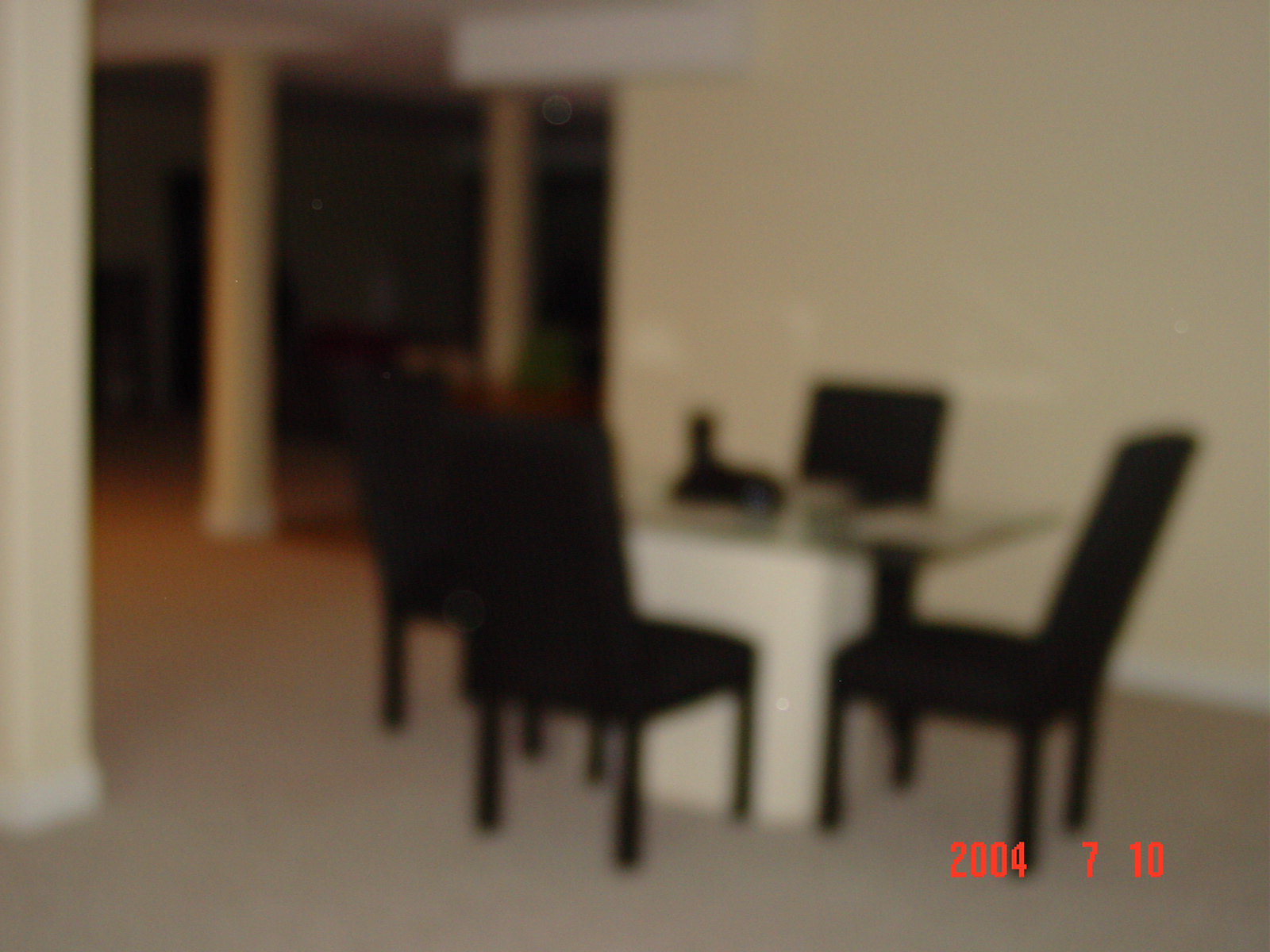This blurry photograph captures a dining room scene with a rectangular table that appears to have a granite top, although the detail is unclear due to the blurriness. The table is surrounded by four black Parson's chairs, their distinctive design standing out even in the lack of clarity. The floor is covered with beige carpet, complementing the pale yellow walls and white trim that enclose the space. In the background, a pair of columns can be seen, possibly marking the entrance to a living room, which remains shrouded in darkness and difficult to discern.